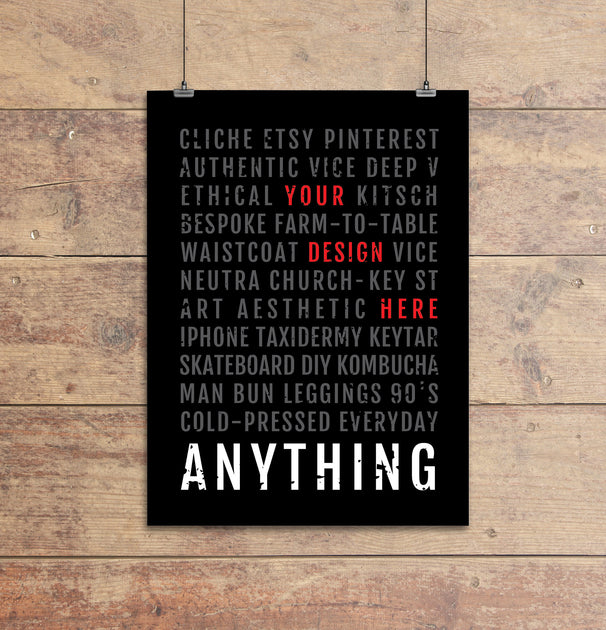The image showcases a square photograph of a black rectangular poster, emphasized by a wooden plank background with light brown hues. The poster, suspended by two black wires clipped to the top left and right, features predominantly gray text, interspersed with white and red words. Central to the poster are the striking red words "your design here," while the bottom showcases the word "anything" in large, bold white capital letters. Surrounding "anything" within the black rectangle are various highlighted words and phrases such as "cliché," "Etsy," "Pinterest," "authentic," "bespoke," "Nutri-Church," "skateboard," "DIY," "kombucha," "man bun," "leggings," and "90s," suggesting a mix of modern and hipster-themed buzzwords. The setting appears to be indoors, possibly an office or bedroom, enhancing the focus on this striking mix of textual elements designed for visual impact.